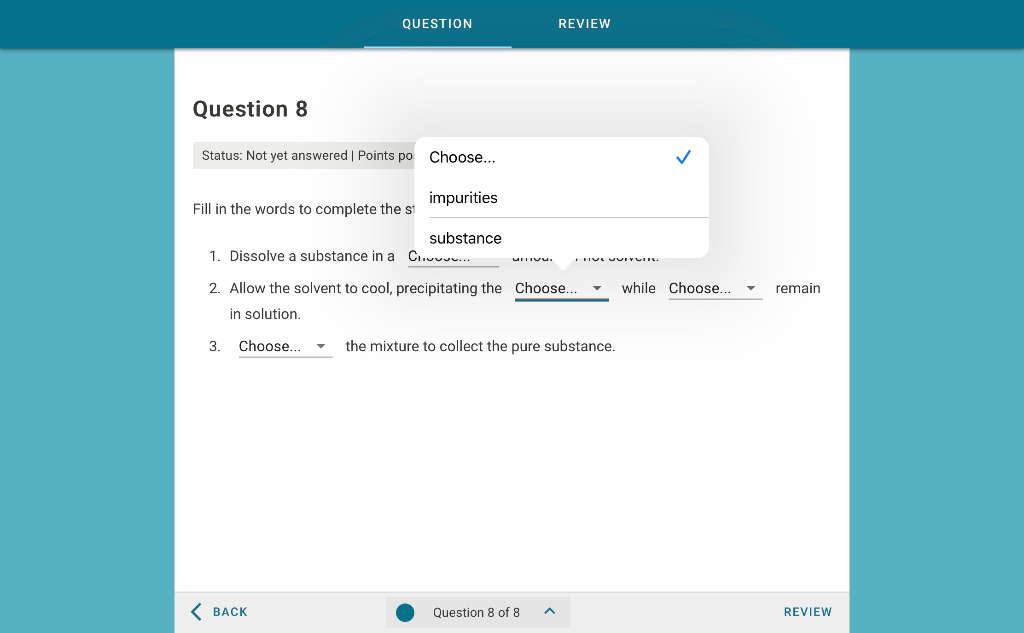**Detailed Caption:**

The screenshot showcases a web page featuring test questions. At the top, a dark green or dark teal navigation bar spans across the screen, with two central tabs labeled "Question" and "Review" in white text. The "Question" tab is underlined in white, indicating it is the active tab. 

Below the navigation bar, the main content area has a white background. Positioned at the top left of this section, the text reads "Question 8" followed by the status "Not yet answered" and the designation "Points: PO." An overlapping box prominently asks users to "Choose impurities in substance, one word per line," obstructing part of the underlying content. 

The blocked section includes a fill-in-the-blank style instruction starting with "Fill in the words to complete the S," which suggests the beginning of a sentence or title. Beneath this, numbered steps guide the user through a process. Step one reads "Dissolve a substance in a," which is partially cut off by the overlapping box. Step two states, "Allow the solvent to cool, precipitating the," followed by a dropdown menu choice, and "remain in solution," with another dropdown menu to select an appropriate word.

The extraneous concluding phrase, "We hope you found this helpful. If you did, please leave a comment. And, if you have any questions, please leave a comment. We'll be happy to answer any of those. Thank you," indicates a supportive and interactive element, though it was not necessary for the descriptive section of the screenshot.